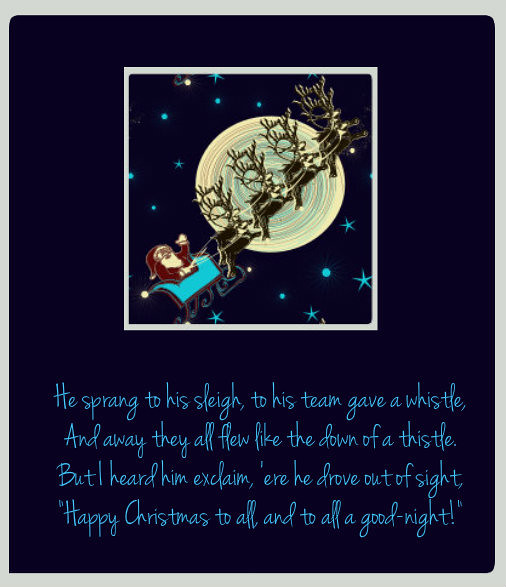The image is a dark blue greeting card with a light gray border, resembling it's placed on a light gray surface. At the top center, there's a square outlined in white containing an illustration of Santa Claus and his reindeer in flight. Santa, positioned in the bottom left corner of the square, is waving with his left hand as his teal sleigh ascends diagonally to the upper right, guided by eight reindeer organized in four rows. The moon, a large yellowish-white circle, creates a luminous backdrop beyond the reindeer, surrounded by teal stars and small blue circles, adding a whimsical touch to the night sky. Below this illustration, covering approximately the lower third of the card, is a four-line excerpt from 'Twas the Night Before Christmas, written in light blue cursive: "He sprang to his sleigh, to his team gave a whistle, and away they all flew like the down of a thistle. But I heard him exclaim, 'ere he drove out of sight, 'Happy Christmas to all, and to all a good night.'" This embellishes the card with a festive and sentimental greeting.